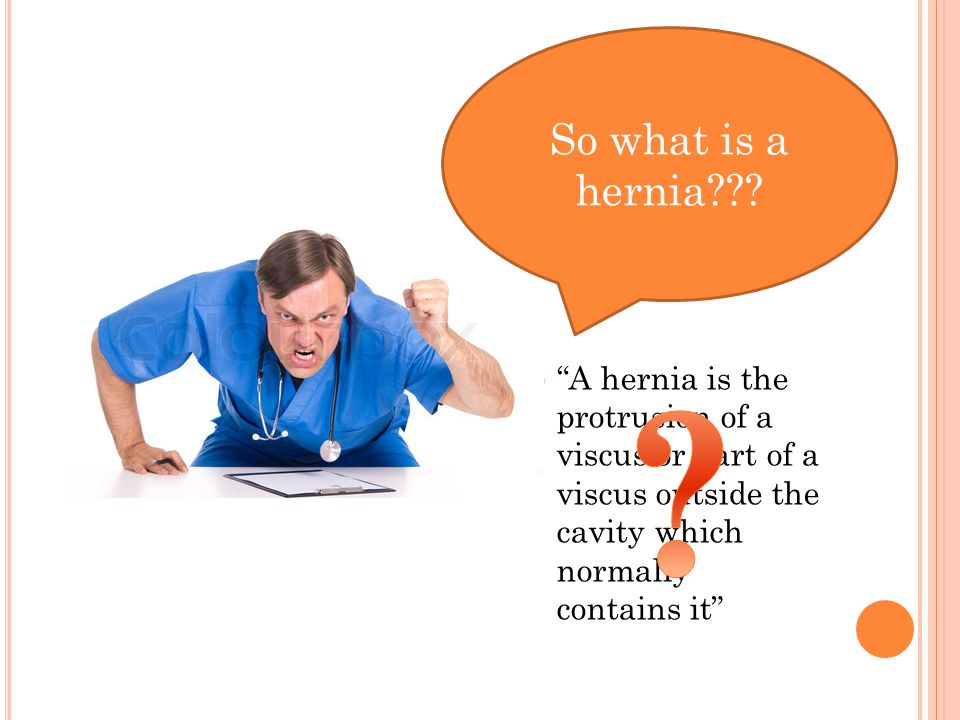The image depicts an angry doctor who has short brown hair and is wearing blue scrubs, a short-sleeved top, and blue pants. A stethoscope with a black cord and silver earpieces hangs around his neck. He is leaning over a table with his left fist raised in the air and his right hand lying flat on the surface. His mouth is open in a furious yell, displaying his teeth. A clipboard with a piece of paper lies on the table in front of him. The background is white. To the right of the image, there is a large orange speech bubble with white letters that ask, "So what is a hernia???" Below this, in black letters, it is explained, "A hernia is the protrusion of a viscous part of the viscous outside the cavity which normally contains it," although some of these words are obscured by a large orange question mark. The lower right-hand corner contains a small orange circle.